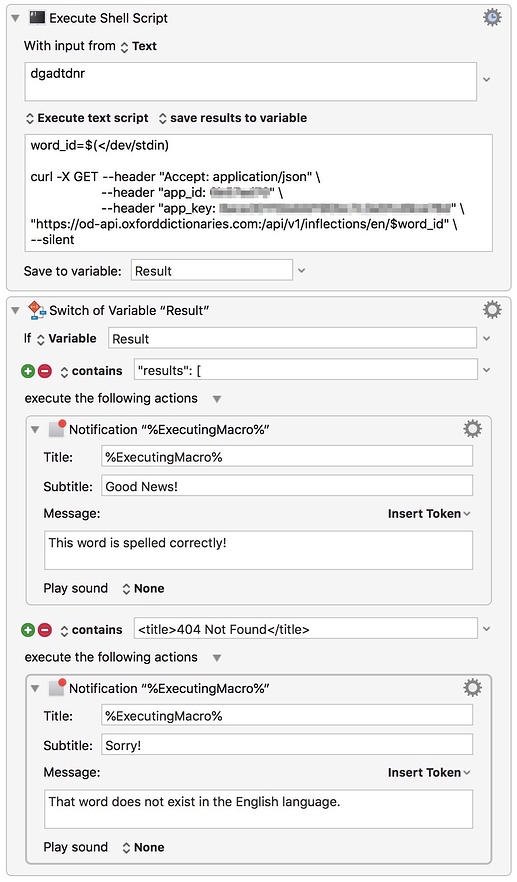The image is a detailed screenshot of an application window designed for executing shell scripts and managing their results. At the very top, there's a programming-related logo followed by the label "Execute Shell Script" and a gear icon on the top right. Below that, there is a section labeled "With input from" with an adjacent text box. 

Further down, the interface features another section titled "Execute Text Script and Save Results to Variable," containing a text box filled with some code. Directly below, it reads "Save to variable: results," followed by a box labeled "Switch to Variable: results." This section includes a "Variable" label and a text box containing the word "results." 

There's a green plus button and a red-minus button, indicating options to add or remove items, with a label saying "Contains results," and a text box containing the word "results."

Following this, there’s a section titled "Execute the Following Actions," succeeded by a box labeled "Notifications" and "Executing Macros." This section also houses fields for "Title" and "Subtitle," each with their own text boxes filled with text. Beneath this, there is a "Messages" section and an associated text box containing some words, followed by an option to "Play Sound."

At the bottom of the image, another segment with a green plus button and a red-minus button is present, with a white text box containing some text. Again, it specifies "Execute the Following Actions" and includes a "Notifications" and "Executing Macro" box. This is followed by sections for "Title" and "Subtitle," each with respective text boxes, and a "Message" section with an additional text box underneath.